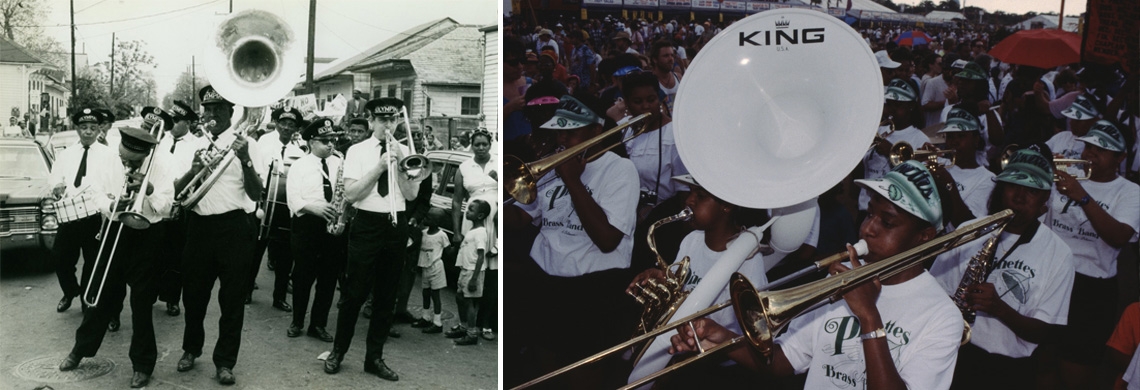This is a wide landscape photograph divided into two sections by a white line, presenting two images of marching bands from different eras. On the left, a black-and-white photograph depicts an older marching band, likely from the late 1960s to early 1970s, given the vintage cars and the attire of black pants, white shirts, and ties. The band members, including a prominent tuba player, are marching down a street lined with spectators and vehicles. On the right, a modern, colorful photograph shows a contemporary marching band, possibly a children's group, wearing white shirts adorned with green lettering and details, and sporting caps or sun visors. The white shirts appear to read "Peanuts Brass Band." The vibrant scene reveals the gold of various brass instruments like tubas, trombones, and French horns played by young musicians. Notably, someone in the crowd holds a red umbrella, suggesting it might be raining. The two images collectively highlight the enduring tradition of marching bands across different generations.